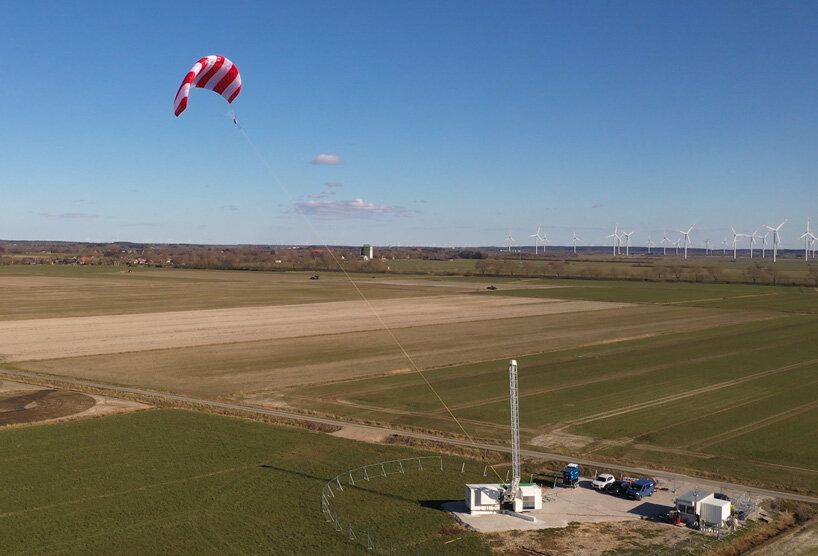In this slightly elevated, drone-like image, a research facility is prominently featured in the middle of an expansive, flat agricultural field. The facility consists of two trailers, one of which is a white utility building with a large metal scaffold-like tower extending from its roof. Attached to this tower by a yellow rope is a red-and-white striped parasail, floating toward the left at about a 45-degree angle, functioning like a kite. A metal chain-link fence encloses this facility, which includes a cement pad serving as a parking area for a few cars.

Connected to a small country road visible on the right side of the image, the land around the facility extends as far as the eye can see, dotted with light greenery and clear of major obstructions. Far in the distance to the right, a wind farm with approximately 30 tall white windmills stands against a clear blue sky with very light clouds, hinting at the facility's potential role in wind research. The scene is bathed in sunlight, suggesting it is late in the evening.